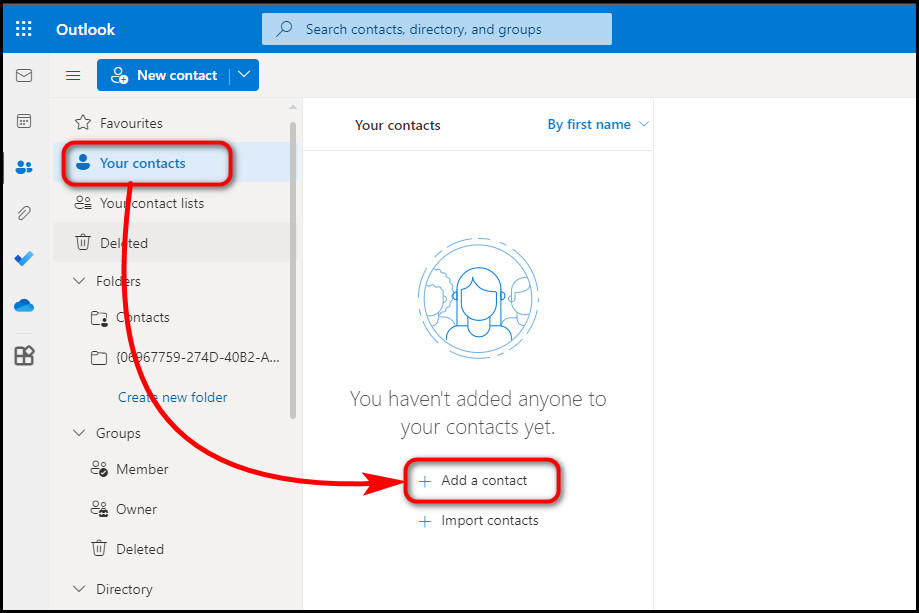The image depicts a screenshot of the Outlook web interface with various UI elements and annotations highlighted for emphasis. 

At the top, against a blue background, is a grid of nine white squares forming a larger square, next to which the word "Outlook" is displayed in white. Below this in the same blue banner, there’s a light blue magnifying glass icon adjacent to the text "Search, Directory, and Groups," all in light blue.

The background underneath progressively turns gray. On the left-hand side is a blue rectangle with the text "No contact" in white. Below, an outlined black star marks the "Favorites" section. Highlighted in blue, denoting a selected state, is the text "Your Contacts," encircled by a red box with an arrow pointing to a different area of the screen.

On the right side, the arrow leads to a section with a blue plus sign and the text "Add a Contact" also enclosed in a red box. Below this, another blue plus sign precedes the text "Import Contacts" in black. Above both options is a message, "You haven't added anyone to your contacts yet."

At the very top of this section, "Your Contacts" is labeled in black. Adjacent to this, the text "By First Name" appears in blue with a downward arrow indicating a sorting option. Further down, under "Your Contacts," there are several labels: "Deleted," "Folders," "Contacts," and "Create Folder" in blue, followed by "Group Members Only," "Deleted," and "Directory" in black.

The screenshot is likely intended to instruct users on managing their contacts within the Outlook platform.